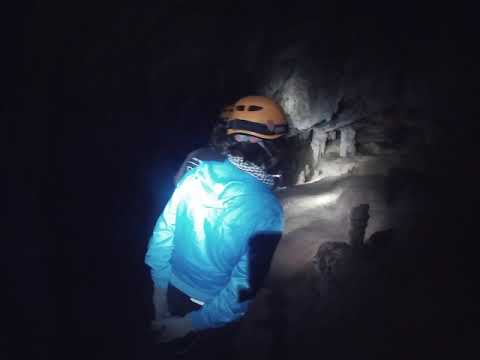The photograph captures the inside of a dimly-lit cave with predominantly dark surroundings, punctuated by limited visible light. It features two individuals in the center: one person with their back turned, wearing a blue jacket and an orange helmet, which seems akin to a construction helmet for protection. The other person, partially obscured, is similarly clad in a black jacket and orange helmet. A scarf is noticeable around the neck of the person in the blue jacket. The cave’s roof and ground are marked by irregular, gray-colored structures, lending a rugged texture to the scene. The edges of the image fade into complete darkness, hinting at the cave's expansive and shadowy interior. Scattered rocks and potentially sand cover the cave's floor, contributing to the overall ruggedness of the environment.